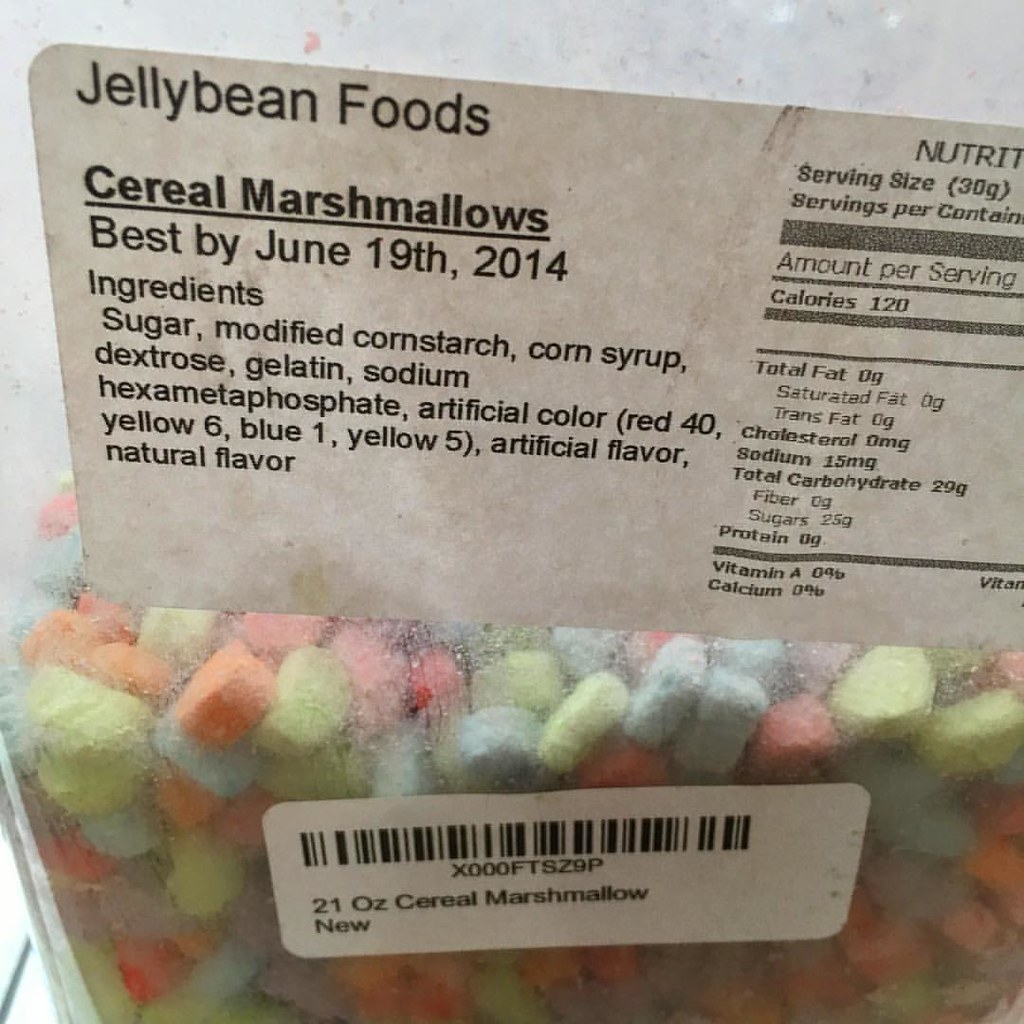This is a detailed close-up photograph of a clear plastic container filled with colorful cereal marshmallows, reminiscent of those found in Lucky Charms. The marshmallows, varying in hues such as light blue, light green, pink, and orange, are scattered below a prominent label occupying the top portion of the image. The label reads "Jelly Bean Foods Cereal Marshmallows" and indicates a best-by date of June 19, 2014. It lists the ingredients: sugar, modified cornstarch, corn syrup, dextrose, gelatin, sodium hexametaphosphate, artificial colors (Red 40, Yellow 6, Blue 1, Yellow 5), artificial flavor, and natural flavor. To the right of the label is a partially visible nutrition guide, specifying a serving size of 30 grams with 120 calories per serving and 25 grams of sugar. The container also features a rectangular sticker towards the lower portion, containing a barcode and reading "21 oz. Cereal Marshmallow New." The background of the image consists of light gray tiled surfaces, adding contrast to the vividly colored marshmallows.